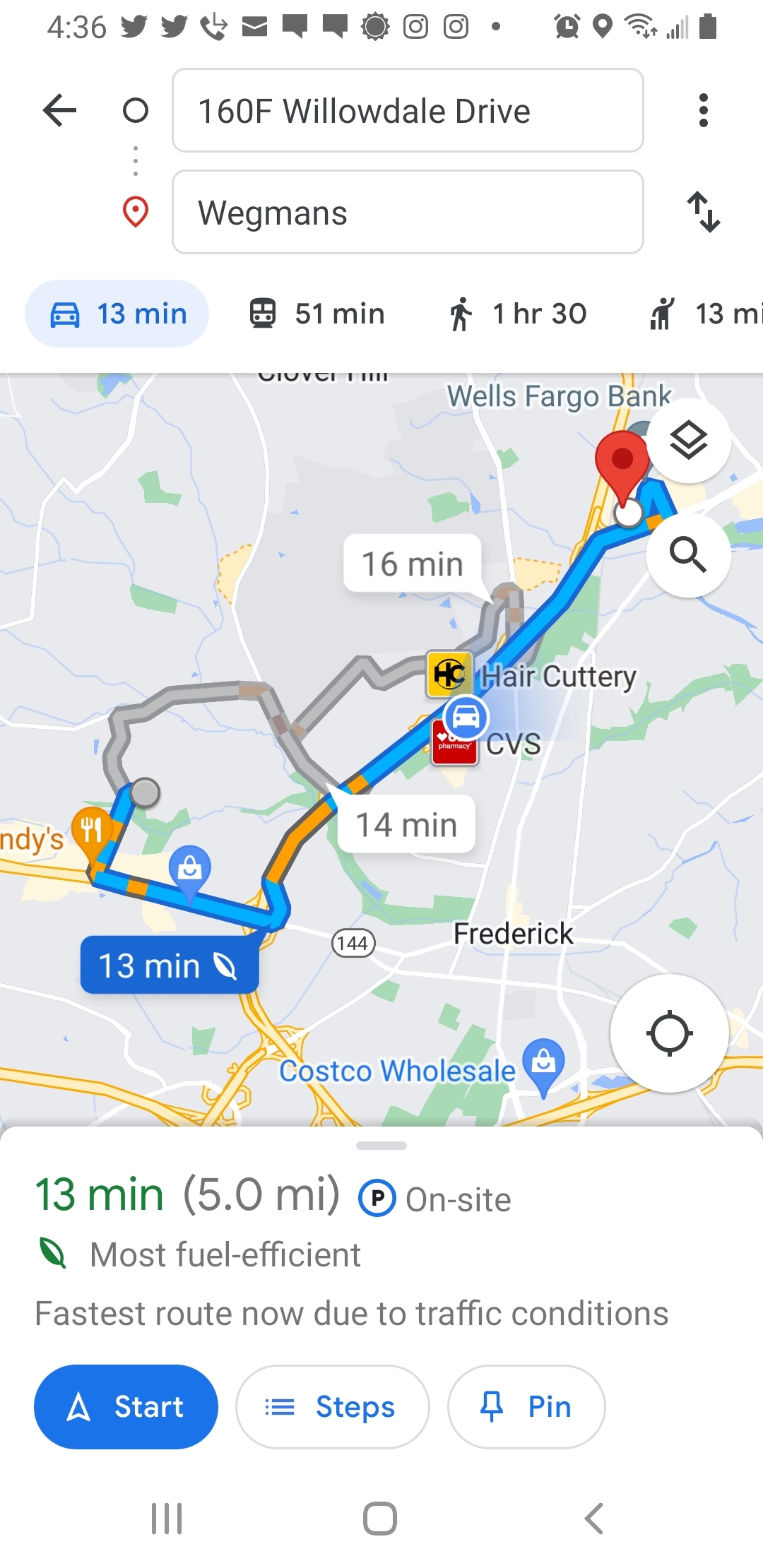This image is a detailed screenshot taken from an Android cellular phone displaying a Maps application, such as Google Maps. The screen shows navigation instructions from the starting location at 160F Willowdale Drive to the destination, Wegmans grocery store. The suggested route, highlighted in blue, is the fastest and most fuel-efficient, taking 13 minutes to cover 5 miles, given current traffic conditions. The map also features noticeable icons and notable landmarks along the route, including Costco, CVS, Hair Cuttery, and Wells Fargo Bank. At the top of the screenshot, various system icons and the current time, 4:36, are visible. Additionally, alternate travel options are listed, such as a 51-minute train ride, a 1 hour-and-30-minute walk, and an indicated distance for hitchhiking. The comprehensive view clearly maps out the quickest path, using both color highlights and traffic indicators.